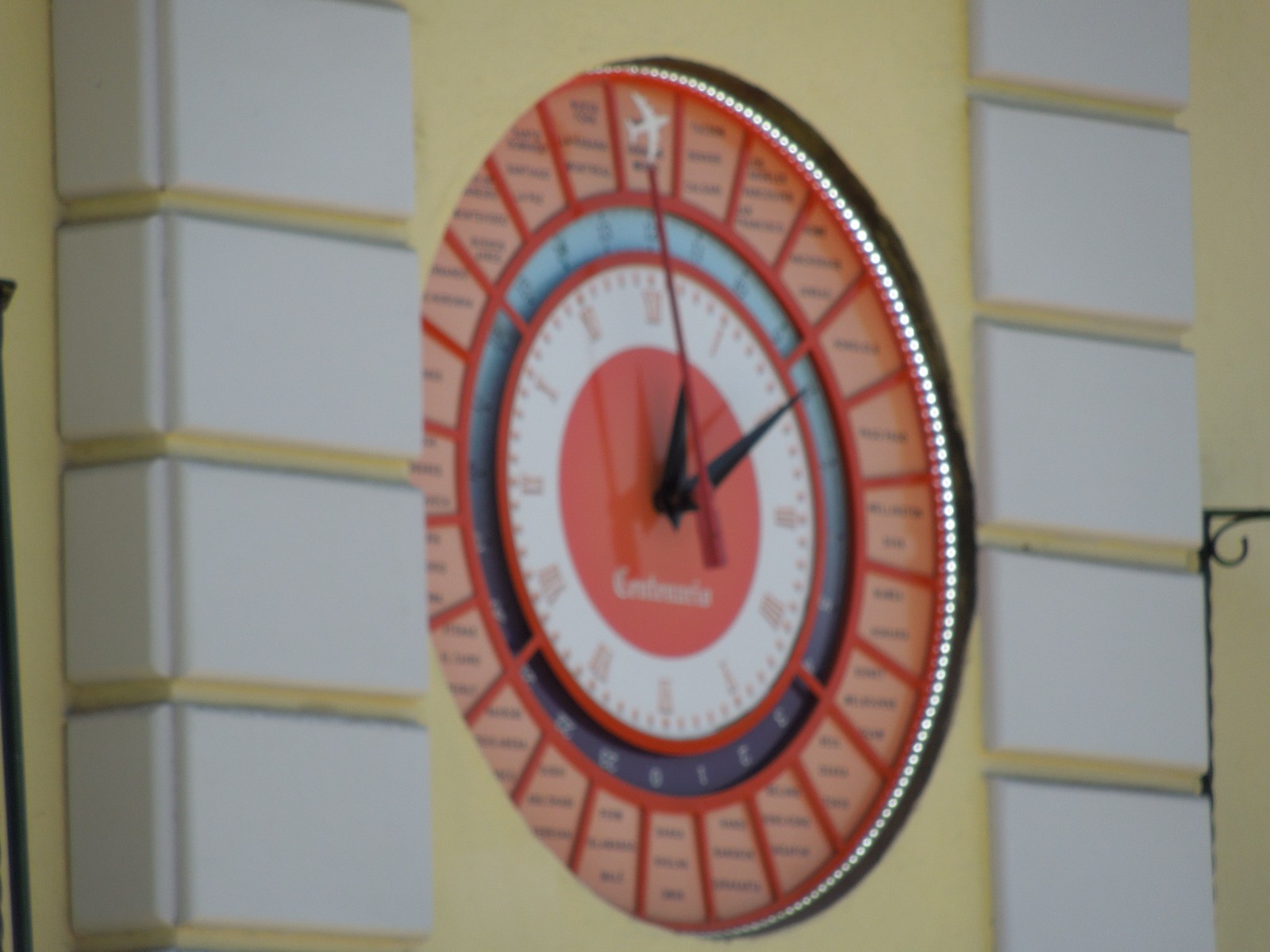In this photograph, though somewhat blurry, one can perceive an outdoor clock mounted on a yellow wall. Despite the lack of sharp details, the clock exhibits a remarkable design with an intricate blend of red and salmon hues. The interior of the clock features a white section complemented by a deep reddish salmon color. Notably, an airplane icon adorns the top of the clock, indicating a possible connection to aviation, potentially suggesting that it is located at an airport or an aviation-related venue. The exact time displayed is indistinct, but it appears to be approximately 12:10.